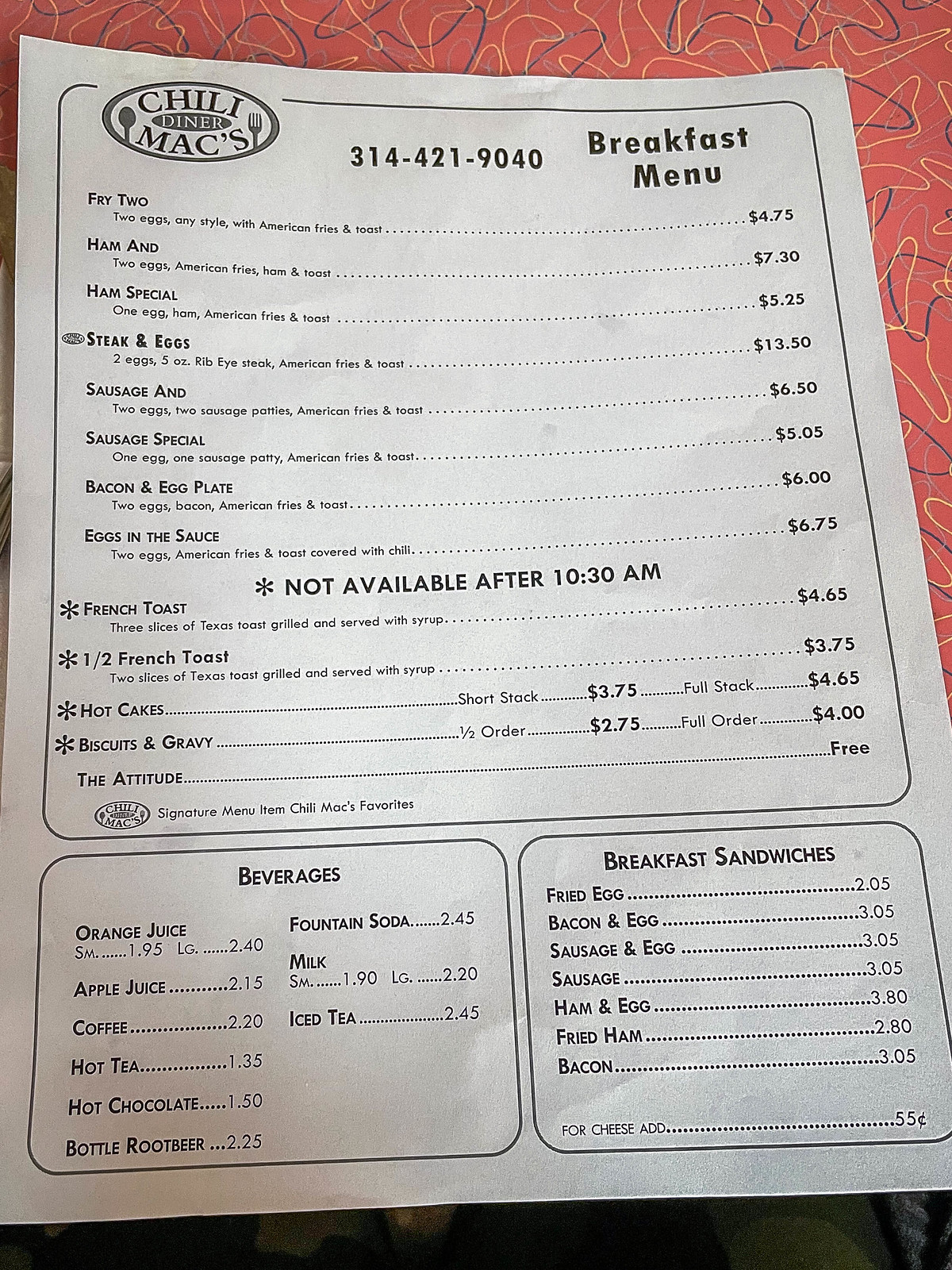In the photograph, a large piece of white paper is placed on a red and blue print tablecloth. In the upper left corner of the paper, the name "Chili Max" is prominently displayed. At the center top, the word "diner" is prominently written, along with the phone number "314-421-9040." Below these details, the heading "breakfast menu" is visible, followed by a list of breakfast items. 

One of the breakfast items listed is the "Ham Special," which includes an egg, ham, American fries, and toast, priced at $5.25. A series of dotted lines extend about three inches to the right, connecting each item to its respective price.

In bold text in the center area, it states, "Not available after 10:30 a.m." Following this, additional breakfast options are listed, including French toast, half French toast, hot cakes, and biscuits with gravy.

In the lower left corner, the "Beverages" section lists drinks such as orange juice, apple juice, coffee, hot tea, hot chocolate, bottled root beer, fountain soda, iced tea, and milk.

Finally, the lower right corner features "Breakfast Sandwiches" with options such as fried egg, bacon and egg, sausage and egg, sausage, ham and egg, fried bacon, and just bacon.